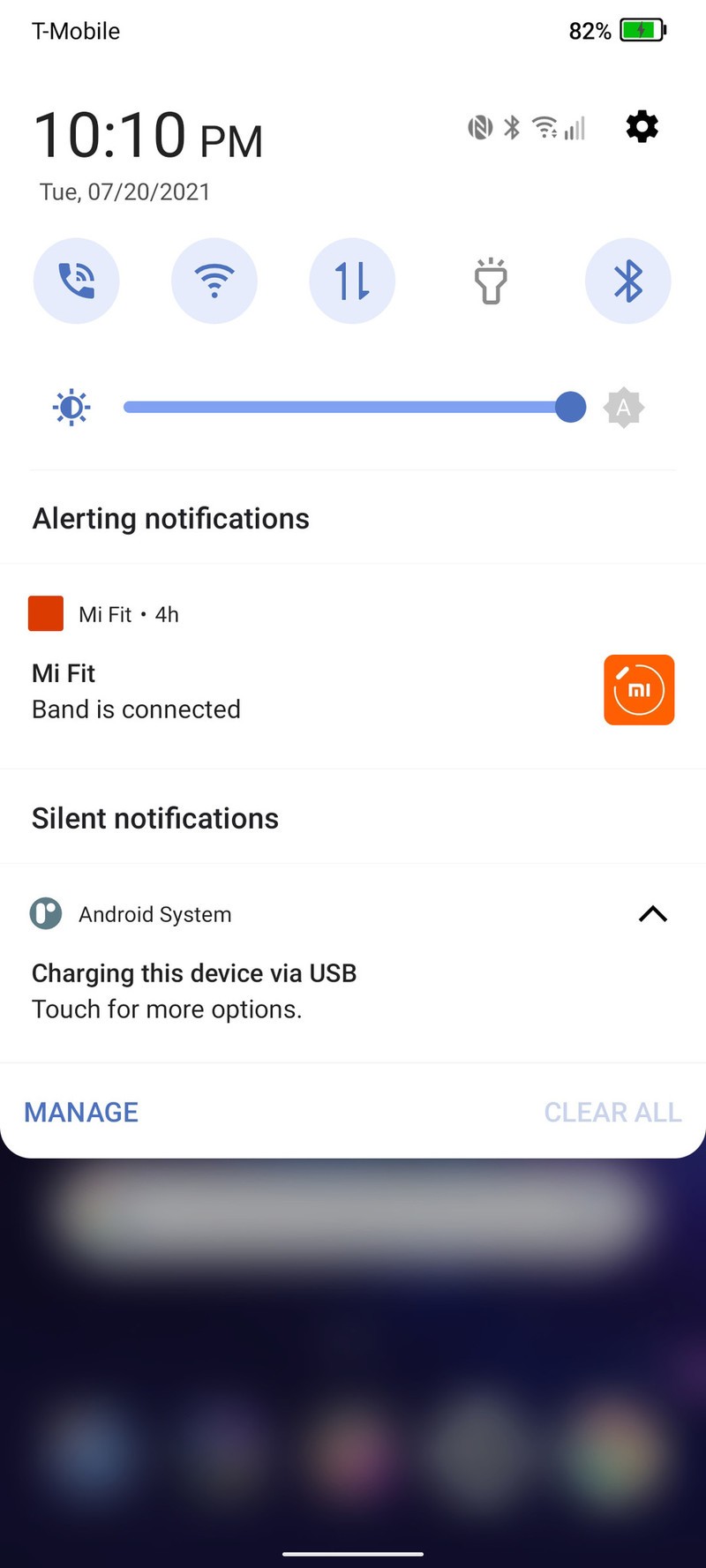Screenshot of an Android phone displaying a pop-up web page with the T-Mobile network provider indicated at the top. The status bar shows 82% battery life with a green charging icon, the current time at 10:10 p.m., and various connection icons including a strange connection icon, Bluetooth, and Wi-Fi. The date is displayed as TUE, 07-20-2021. Below the date are icons for phone call, Wi-Fi, and transmit status with pale blue backgrounds and dark blue icons, followed by a flashlight icon against a white background and another Bluetooth icon in a blue circle. A brightness slider, fully dragged to the right, is visible below these icons.

Further down, the notification panel has an "Alerting Notifications" section with a small orange square for MyFit and the message "MyFit: The band is connected," accompanied by the MyFit orange icon. The "Silent Notifications" section below includes an indeterminate icon and the Android system message "Charging this device via USB" with a prompt to "Touch for more options." The options "Manage" and "Clear all" are visible, though "Clear all" is not highlighted. The blurred background image of the cell phone screen shows five icons at the bottom.